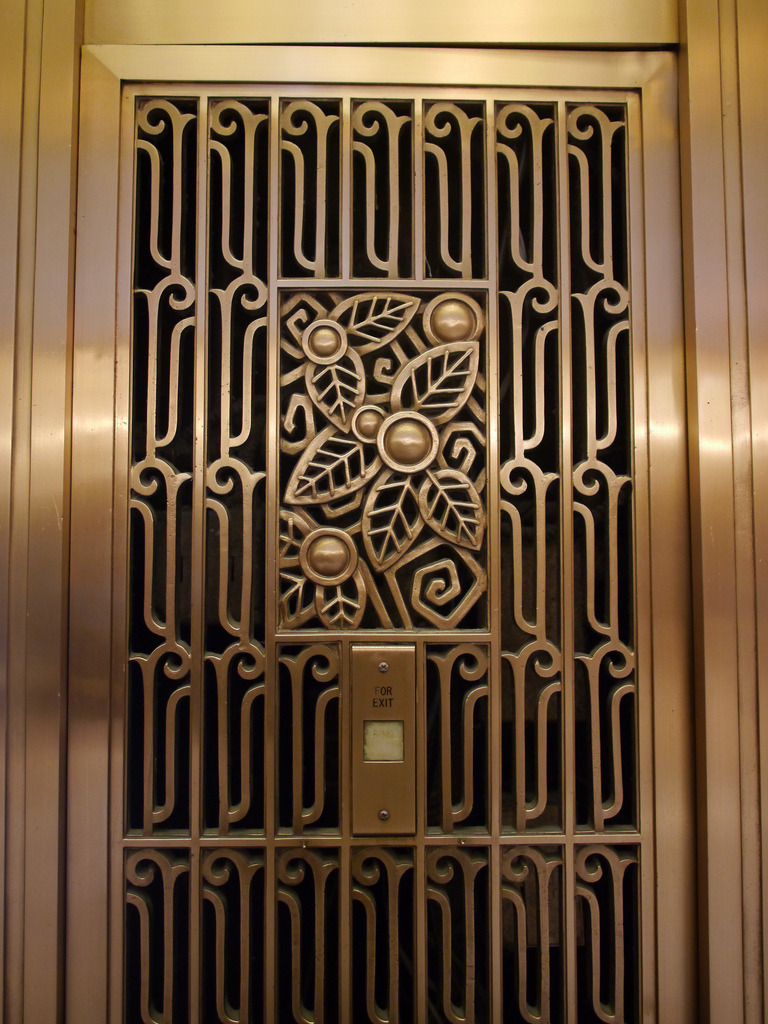This image showcases a gold-colored security door, likely made of metal, featuring intricate Art Deco design elements. The door is adorned with vertical and curlicue patterns, and it also includes a central tall rectangle that houses a stylized flower and leaf design, all in gold. Below this decorative panel, there’s a prominent small white button labeled "for exit" that appears to be a bell or push-button, surrounded by screws. Additionally, the door frame and surrounding area are also gold-hued with circular and trumpet-like ornamental accents, contributing to its opulent and possibly historical aesthetic, suggesting it could lead to an upscale apartment, hotel, or bank.